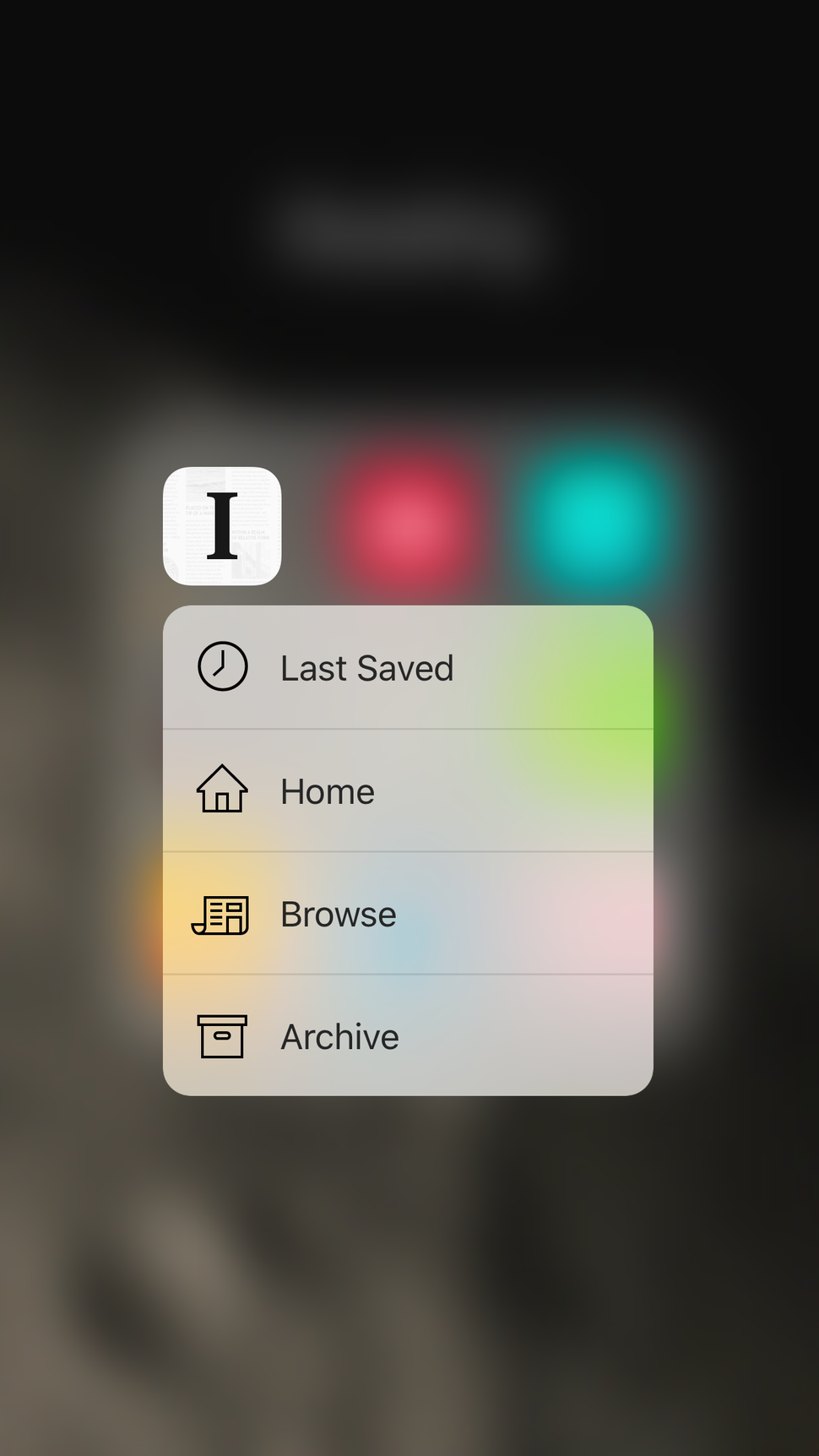The image captures a phone screen where a folder containing multiple apps has been tapped, causing a semi-transparent overlay to appear. At the top of this overlay, partially obscured text begins with "I" and quickly blends into the background. The semi-transparent overlay forms a near-perfect square, allowing the interface elements below it to be faintly visible. Centrally positioned within this square are four distinct buttons labeled "Last Saved," "Home," "Browse," and "Archive." Each label is accompanied by a small icon adjacent on the right side. The background colors of the screen remain faintly visible through the transparency of the overlay, offering a subtle, yet perceptible, hint of the underlying interface colors.